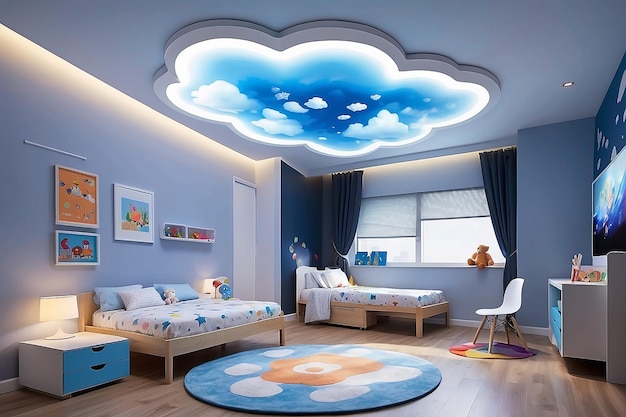The image depicts a hyper-realistic, AI-generated design of a spacious and modern children's bedroom. The room features a sleek wooden floor and is softly lit, primarily by a large, cloud-shaped light fixture on the ceiling, which projects a serene sky with clouds, enveloping the space in gentle illumination. At the center of the room lies a circular rug with a sky-blue background, white clouds, and an orange flower-like design.

The furniture arrangement includes a twin-size bed situated against the far wall beneath a wide window framed by plain grayish-blue curtains. Adjacent to this bed is a white chair and a small white bureau with blue drawers. On the left side of the room is a double bed positioned lengthwise along the wall, accompanied by a small set of drawers serving as a side table with a white lamp on top. Decorative elements such as childlike pictures and a teddy bear on the windowsill enhance the room’s youthful charm. The overall aesthetic is modern, clean, and thoughtfully arranged to highlight the design elements, making it an ideal showcase for children's bedroom furnishings.